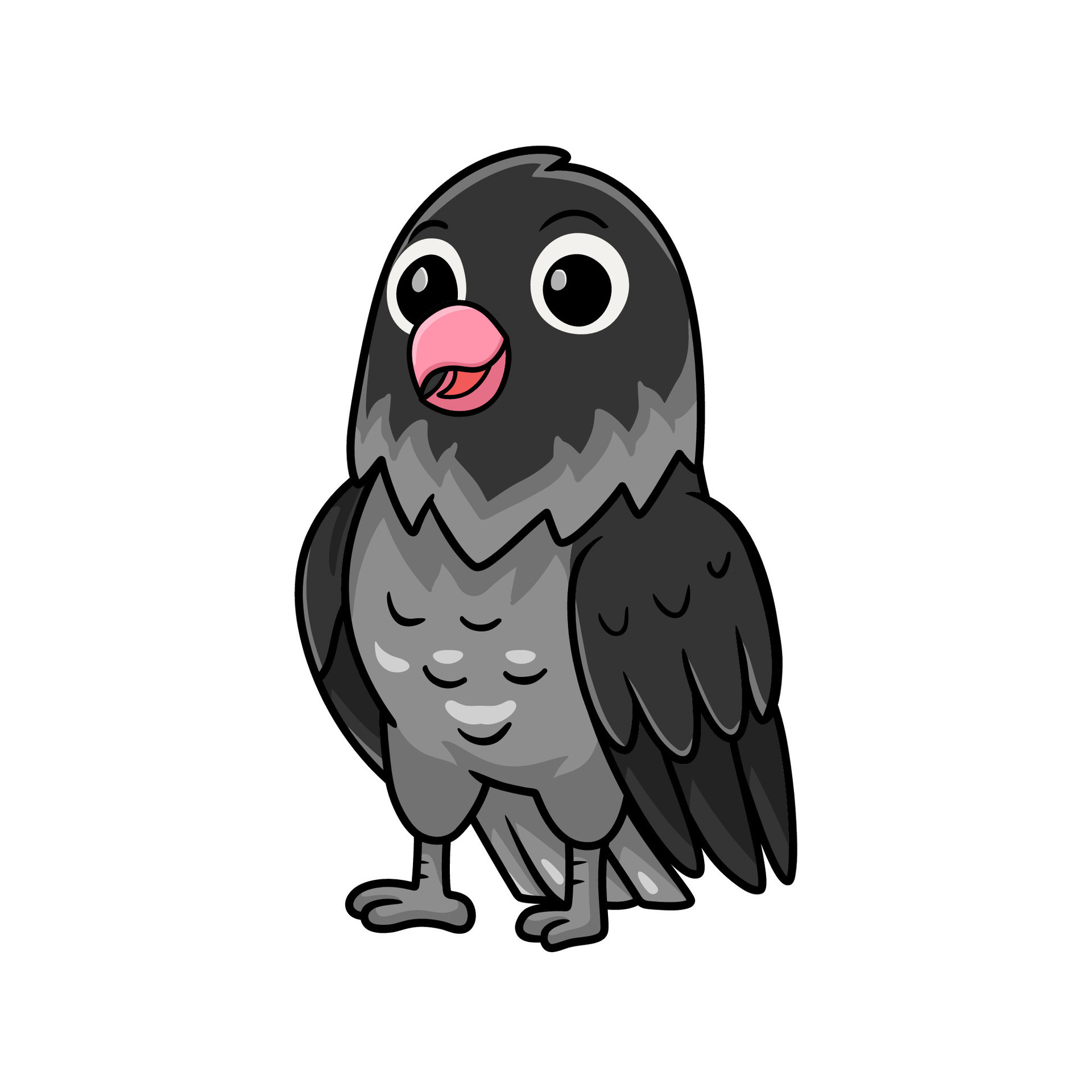This is a detailed two-dimensional cartoon image of a parrot set against a white background. The parrot features a deep gray head and wings, with a medium gray chest adorned with little black curved lines and lighter curved lines indicating feathers. Its tail feathers are light gray with white dots, and the light gray legs and claws accentuate the uniformity in color. The parrot's face includes large, expressive white eyes that appear to be smiling, along with a pink beak and a lighter pink tongue. Dark gray outlines define its features, and the lower part of its head transitions from dark gray to medium and light gray, almost resembling a beard. Its distinctive eyebrows are simply indicated by small lines. The bird sports three toes on its right foot, two on its left, and displays three protruding tail feathers. The overall design, with exaggerated proportions and meticulous detailing, suggests that this cartoon parrot could be a mascot or logo, though no specific affiliation is evident.